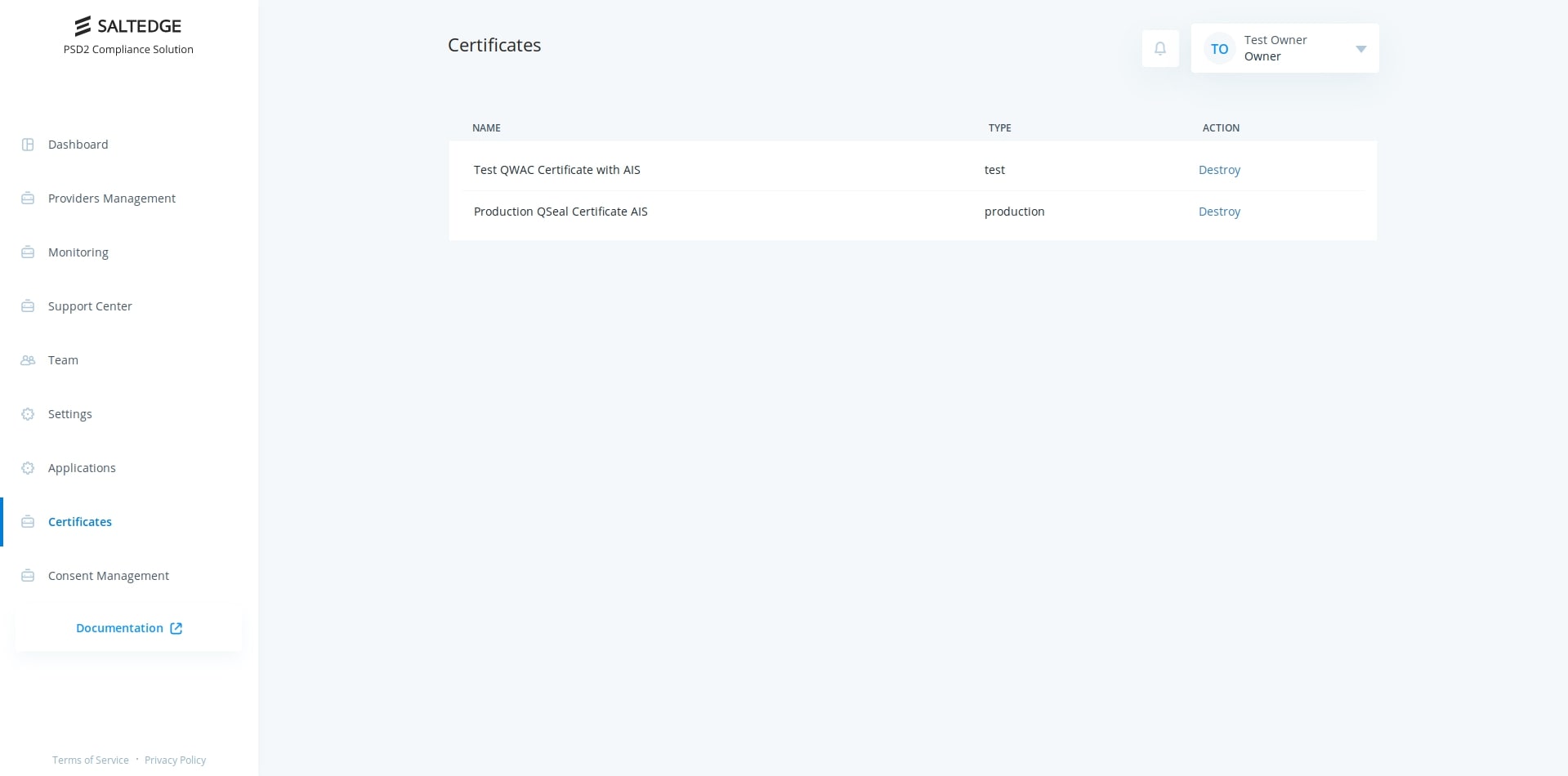The website's interface is predominantly dark blue and grey, featuring a structured layout. At the top of the webpage, the heading "Certificates" is prominently displayed. On the far left of the top bar, there is a white square containing a grey bell notification icon. Adjacent to it, there is a bluish-grey rectangle housing a grey circle with cyan blue text reading "TO" and the phrase "Test Owner" to its right. Below this, the designation "Owner" is written in bold black text, accompanied by a grey drop-down arrow on the right side of the rectangle.

Further down, there is another rectangular section. To the left of this rectangle, within the "Name" column, it lists "Test QWAC Certificate" in uppercase with capitalized initials, followed by "Production QSEAL Certification AIS PQ," also in uppercase with capitalized initials. To the right, in the "Type" section of the rectangle, the entries are "Test" and "Production" on the first and second lines respectively. Lastly, under the "Action" section located outside the rectangle, "Destroy" is written in blue text for both entries.

On the left side of the webpage, a vertical column displays the company logo at the top, which consists of three black lines of varying thickness and orientation. Below the logo, the company name "SALDGE" is written in uppercase, followed by "PSD2 Compliance Solution," with the 'P', 'D', 'C', and 'S' capitalized. Below this, a series of clickable buttons are arranged vertically, labeled "Dashboard," "Providers and Management," "Monitoring," "Support Center," "Team," "Settings," and "Applications." The button labeled "Certificates" is highlighted in blue, indicating it is currently selected. Underneath these buttons, "Consent Management" is listed (not highlighted in blue), followed by "Documentation" which includes a square icon with a blue arrow pointing to the right.